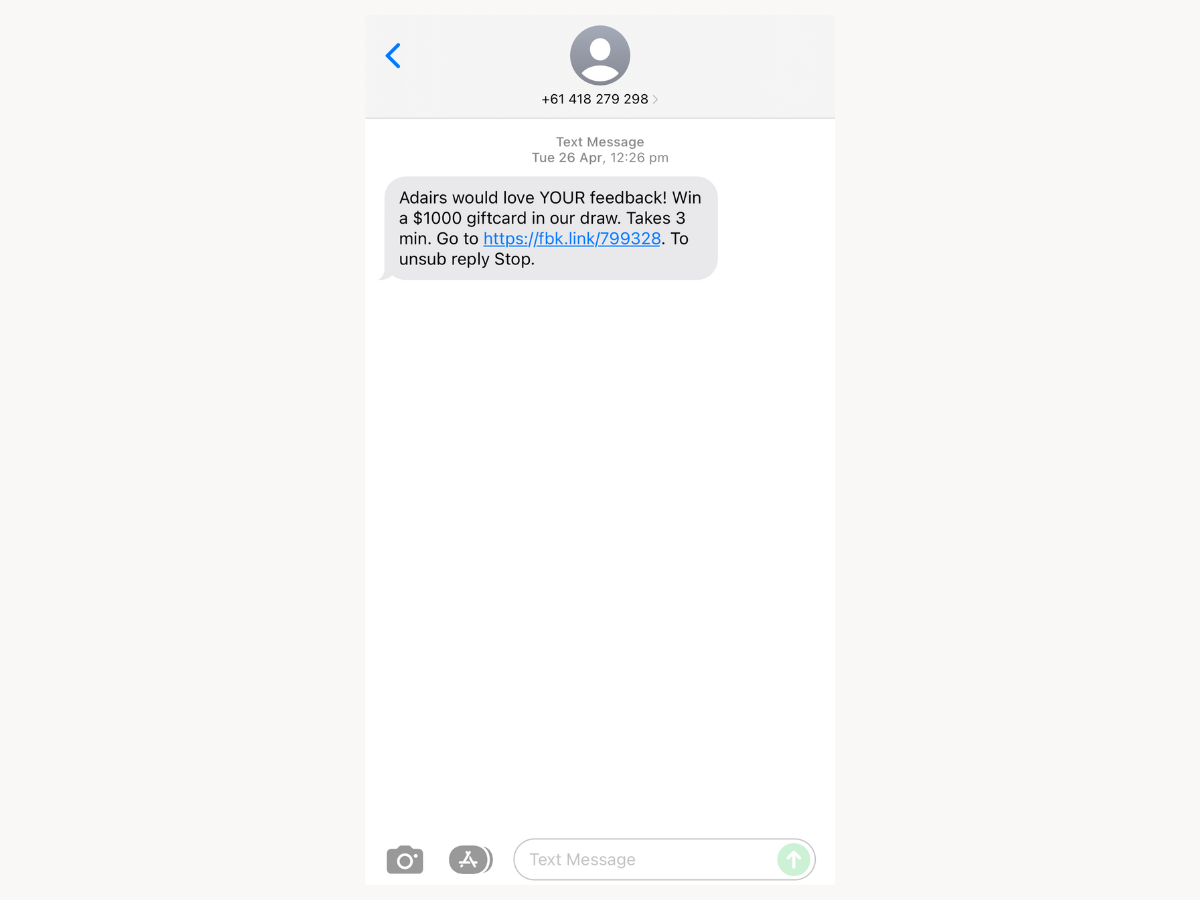The image shows a screenshot from a smartphone displaying a potentially foreign phone number at the top, associated with a generic profile picture. Below, in a white column under the "Messages" app, the timestamp reads Tuesday, April 26 at 12:26 PM. The text message content is portrayed in gray text against a gray background and reads: "I DARES WOULD LOVE YOUR FEEDBACK. WIN A $1,000 GIFT CARD IN OUR DRAW. TAKES 3 MINUTES. GO TO HTTPS://FEEDBACK.LINK//799.328. TO UNSUBSCRIBE, REPLY, STOP." The remainder of the image is primarily white, emphasizing the clean and minimalistic design. At the bottom of the screenshot, standard messaging app icons are visible, including a camera icon, an 'A' within a circle, and a reply text box labeled "Text Message" with rounded edges. To the right of the text box, there's a muted green circle featuring a white arrow pointing upward.